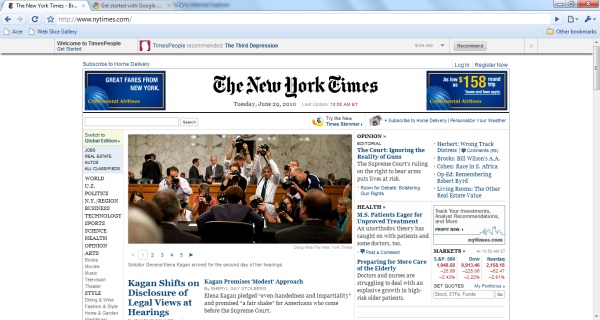The image shows the front page of the New York Times website, dated Tuesday, June 29th, likely from the year 2012. The top of the page features two blue advertisements in the corners, likely for an airline, promoting "Great fares from New York" with prices starting as low as $158. The "New York Times" logo is prominently displayed in the center.

In the middle of the page is a significant news photograph capturing a person, presumably Elena Kagan, standing in front of Congress. The caption suggests this is related to Kagan's stance on the disclosure of her legal views during hearings. The image is taken from behind, showing Kagan facing a swarm of photographers.

To the left of this image, there are clickable sections labeled U.S. Politics, New York, Technology, and Sports. On the right side of the page, there are headlines discussing various issues such as the Supreme Court's stance on gun laws, the healthcare system, and unproven treatments for inmate patients. The overall layout represents the typical structure of the New York Times homepage, offering easy navigation through multiple news categories.